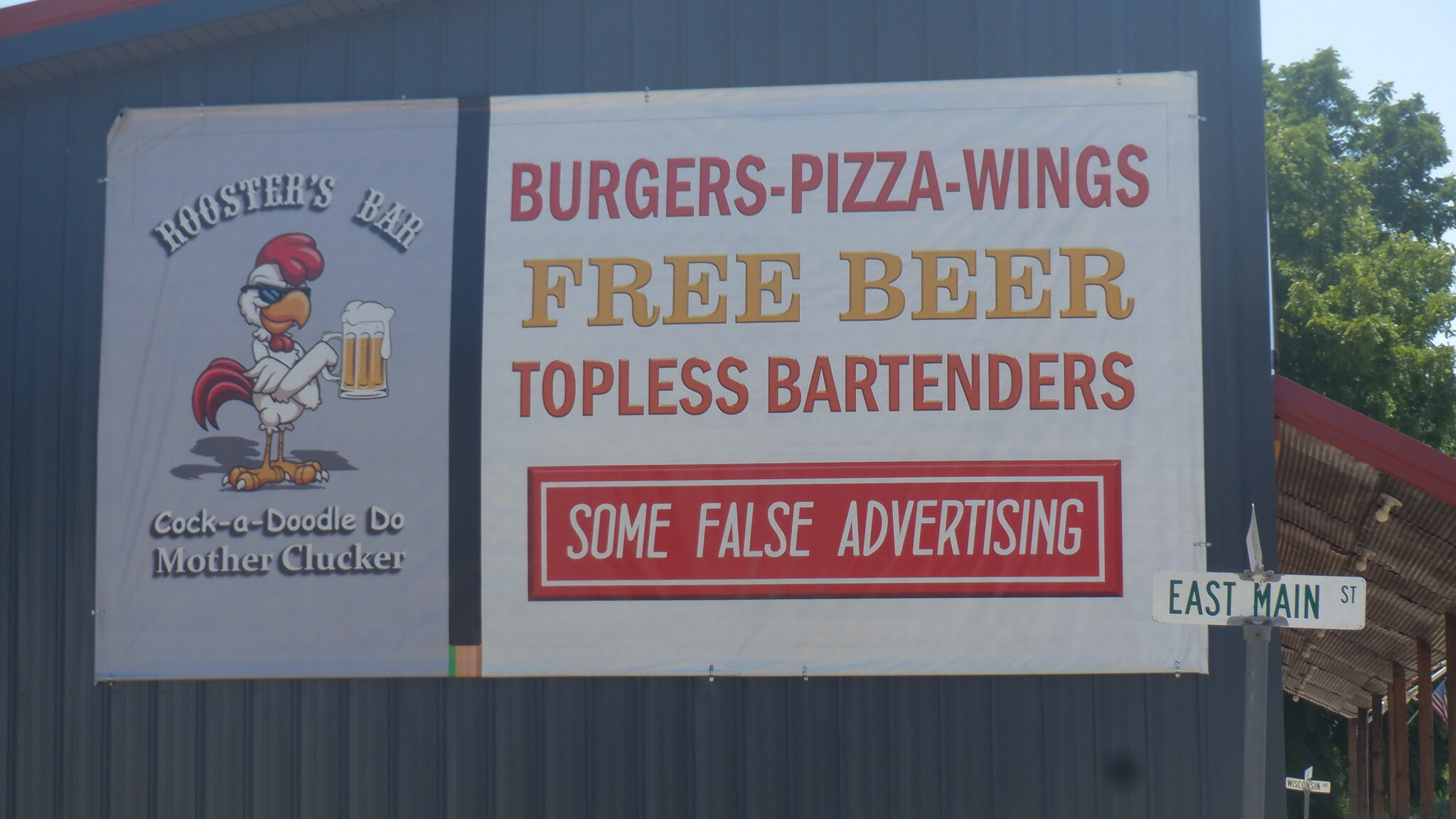This color photograph presents a detailed close-up view of an advertisement mounted on the side of a slate-gray building. Dominating the left side of the ad is a vibrant cartoon depiction of a rooster standing upright, clutching a mug of frothy beer. The establishment's name, "Roosters Bar," is prominently displayed.

On the right side of the photo, the background reveals elements of the surrounding environment: at the very top corner, there are glimpses of green tree foliage contrasting with the urban setting. Below the trees, a red roof is partially visible, which appears to belong to another building or perhaps an awning of the same establishment.

The advertisement's right section features bold, enticing text that lists the bar's offerings: "Burgers, Pizza, Wings, Free Beer, Topless Bartenders." However, humorously undercutting the promotional statement, the phrase "Some False Advertising" is noted below, adding a tongue-in-cheek disclaimer. The juxtaposition of whimsical illustration and cheeky text captures attention and evokes a playful vibe.